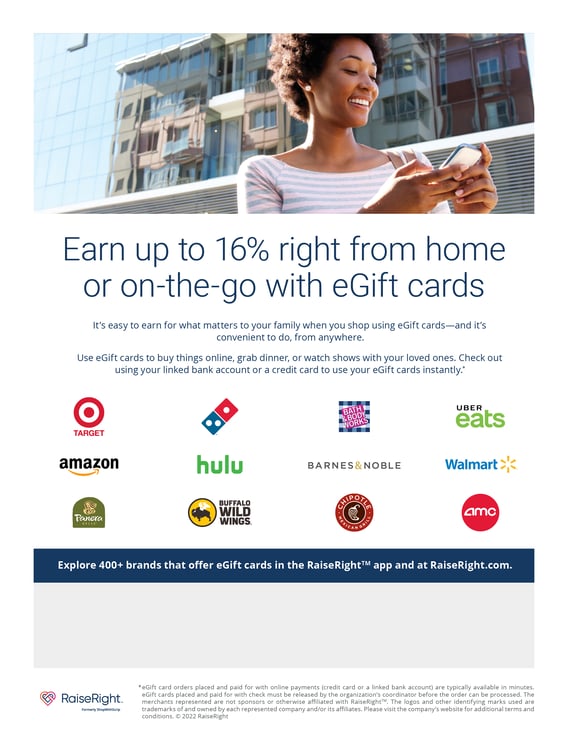This promotional website image showcases a platform that allows users to earn rewards with e-gift cards. The top section of the page features a photograph of a smiling woman with curly black hair, wearing a striped shirt in either white and gray or pink and gray. She is standing outdoors between buildings and is looking at her phone. Overlaying this picture is text that reads, "Earn up to 16% right from home or on the go with e-gift cards. Easily earn for what matters to you and your family when you shop using e-gift cards. It’s convenient to do from anywhere."

Further text explains how users can use e-gift cards to make online purchases, grab dinner, watch shows with loved ones, and check out using linked bank accounts or credit cards instantly. The image also displays various logos of popular retailers and services, including Target, Amazon, Panera, Buffalo Wild Wings, Hulu, Domino's, Bath and Body Works, Barnes & Noble, Chipotle, AMC, Walmart, and Uber Eats, indicating the wide range of options available for e-gift card use.